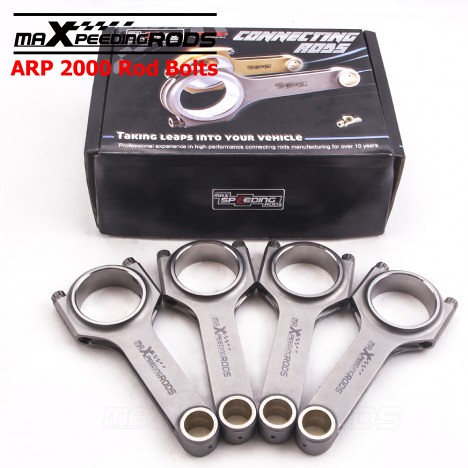This full-color advertisement showcases a set of four ratchets, neatly aligned side by side, accompanied by a sleek black carrying case. The ratchets are identified as MA Expedia connecting rods, specifically designed for automotive use. Each rod is secured with ARP 2000 rod bolts, known for their exceptional strength and reliability. The compact black box, likely measuring around 3 to 4 inches in both width and height, complements the set with both convenience and portability. The image conveys a professional and high-quality impression, ideal for automotive enthusiasts or professionals looking for reliable tools.